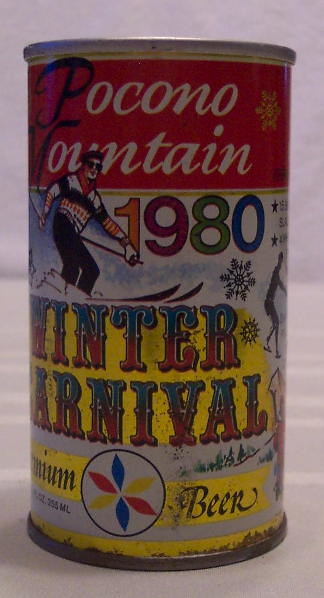This is a color photograph of a vintage beer can, showing signs of rust, especially towards the bottom. The can is smoothly rounded with a lip at the top that has a gold hue. At the top of the can, there's a red banner that reads "Pocono Mountain," where the 'P' in Pocono and the 'M' in Mountain are in black, while the rest of the letters are in white. Below this, there is an illustration reminiscent of pop art, depicting a skier with clown-like makeup, surrounded by stylized snowflakes. This design celebrates the "1980 Winter Carnival," with the year displayed in various colors and the event name in a two-tone blue and red circus font. At the bottom of the label, there's a gold area with the words "Premium Beer," flanked by a multicolored rosette design. This item is photographed on a white surface with a white background. The can appears to have been specially produced for the 1980 Winter Carnival in the Pocono Mountain area.